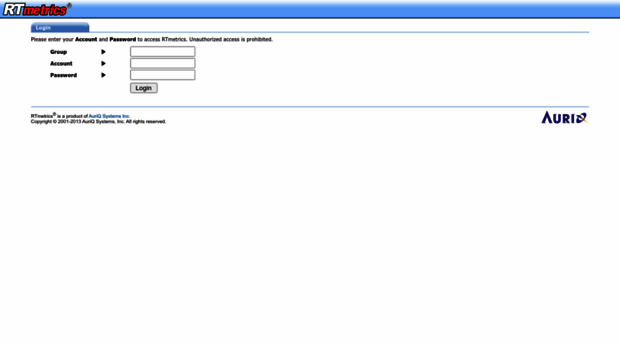The image depicts a computer screen with a user interface for accessing RT Metrics, a service provided by Oracle Systems Incorporated. At the top of the screen, a light blue banner gradually fades into white. Prominently displayed on this banner is the text "RT" in large white letters with a gray outline, followed by the word "metrics" in red with a gray outline. Below the banner, a thin gray line separates the header from the rest of the content. 

A tab labeled "login" is visible just beneath this line. The screen instructs users to "Please enter your account and password to access RT metrics. Unauthorized access is prohibited," though the image quality is notably fuzzy. Below this message, the label "Group" appears in bold black font with a downward-facing arrow icon next to it, followed by a blank search bar. 

Further down, the labels "Account" and "Password" are displayed, each accompanied by a small black arrow and blank search bars for input. There is also a "Login” button present for user authentication. 

At the bottom of the screen, there is a notice stating "RT metrics is a product of Oracle Systems Incorporated. Copyright 2001-2013. Oracle Systems Incorporated. All rights reserved." In the lower right corner of the screen, the acronym "A-U-R-I-O" appears in blue text.